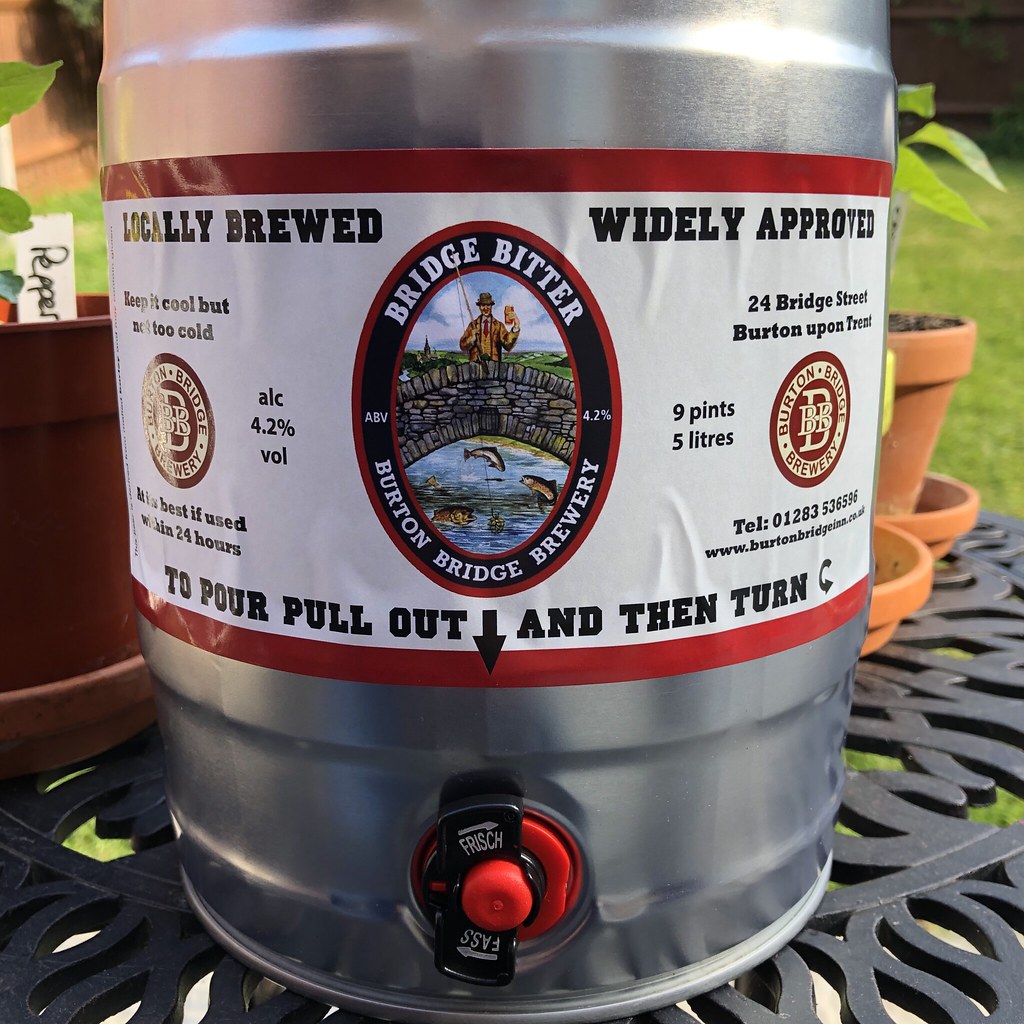The photograph depicts a small, pristine stainless steel keg of beer prominently labeled "Bridge Bitter" from Burton Bridge Brewery. The metallic keg features a white label encircled by red horizontal lines at the top and bottom, bearing the brewery's logo in the center. The logo, an oval design, showcases a fisherman on a stone bridge with fish jumping beneath him. The label text includes "locally brewed, widely approved", an alcohol content of 4.2%, and the capacity of 9 pints or 5 liters. Additional details include the brewery’s address, 24 Bridge Street, Burton upon Trent, a telephone number (01283 536596), and the website (www.burtonbridgein.co.uk).

The keg is fitted with a red spout marked with instructions: "To pour, pull out, and then turn," along with guidance to keep the contents cool but not too cold and to consume within 24 hours for the best quality. The keg rests on a black outdoor wire patio table, surrounded by small potted plants and a grassy lawn in the background, indicating an outdoor setting perfect for enjoying a locally brewed beverage.